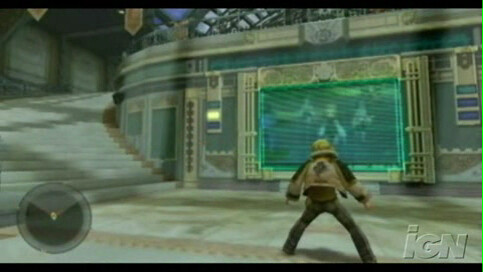The image is a screenshot from a video game, likely captured from a review by IGN, as suggested by the watermark present on the bottom right corner of the screen. At the center-right of the image stands a character, viewed from behind, positioned in front of a screen embedded in a wall with art deco decorations. The character, who has blonde hair, is dressed in a brown, baggy jacket over a brown shirt, paired with black jeans. They are standing with their legs spread wide and arms slightly extended, adopting a wide stance as if ready for action. Directly to the left of the character is a wide, curved staircase with no railing, which ascends to a higher platform. Above this staircase hang a few banners, and parts of a second-floor railing are visible. On the game interface, the bottom right corner features a circular indicator with an arrow, and partially depleting segments, possibly showing the direction the character is facing or some in-game status indicator.